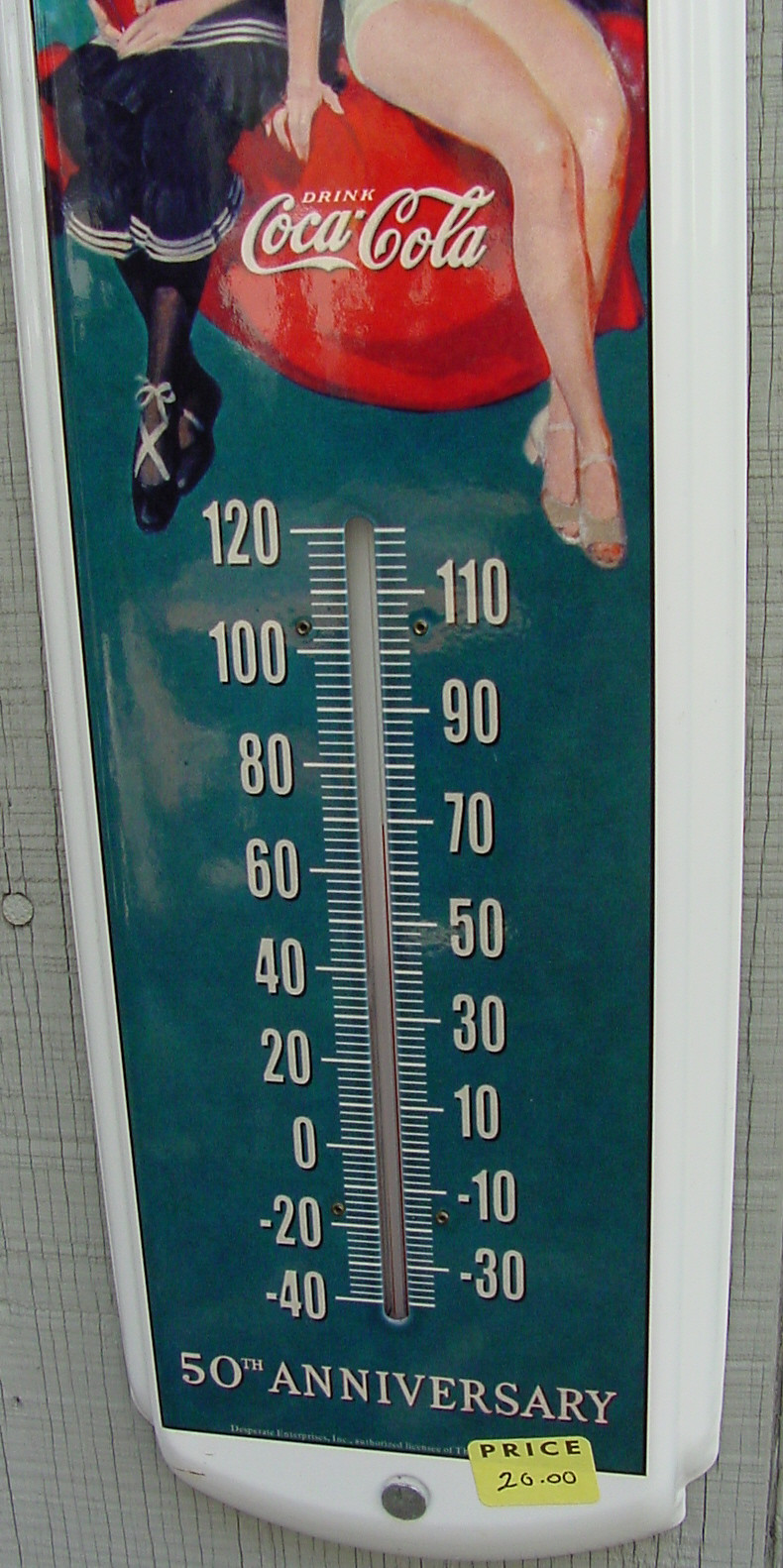This rectangular photograph features an outdoor thermometer with a dark teal hue. Although the top portion of the thermometer is cut off, the lower section remains visible, displaying intricate details. Prominently featured on the thermometer is a vintage Coca-Cola advertisement in red with white lettering, showcasing two women in a nostalgic setting. The woman on the left dons a blue and white skirt, complemented by black leggings and black ballet flats adorned with white laces. In contrast, the woman on the right sports white short shorts and silver heeled sandals, her toes peeking through the open design of the approximately one to two-inch heels.

The thermometer, celebrating Coca-Cola's 50th anniversary, is marked with numerals in white, ranging from -40 to 120 degrees Fahrenheit. A white outer rim encases the thermometer, which is set against a similarly white background. Adding to its vintage charm is a yellow price tag affixed to the bottom right corner, indicating a sale price of $20. This nostalgic Coca-Cola thermometer encapsulates a piece of history in both design and function.